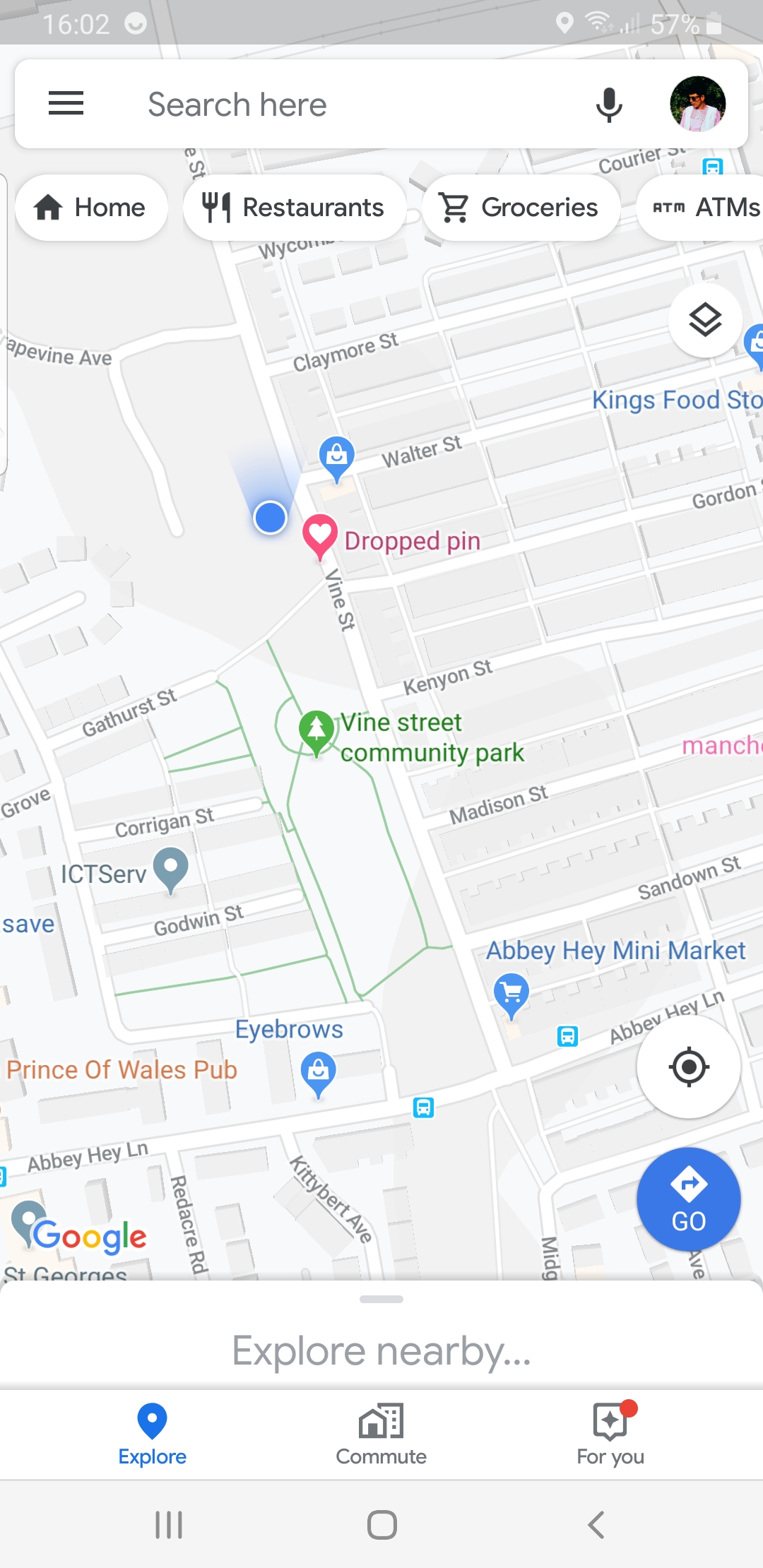A detailed nighttime screenshot of Google Maps on a smartphone screen at 16:02, showcasing various interface elements and a user interface. The top status bar displays a Wi-Fi icon and signal strength with 204 signal bars, a battery life at 57%, and the current time. Below the status bar, a search field appears with a hamburger menu on the left, a microphone icon on the right, and a user icon photo of a thoughtful-looking male in sunglasses, a pink shirt, and a white vest.

The main map interface reveals a location pin dropped amidst an area with visible trees and assorted shopping options. Above the map are functional buttons for Home, Restaurants, Groceries, and ATMs, enabling quick access to these categories. Beneath the map interface lies the "Explore Nearby" section, followed by three tabs: Explore, Commute, and For You. The Explore tab features a map icon with a dropped pin, the Commute tab shows an icon of buildings, and the For You tab has a speech bubble with a red dot in the upper right corner. At the very bottom, the typical smartphone navigation bar is visible.

The map suggests a UK location, highlighting streets named Vine Street, Canyon Street, Gather Street, and Abbey Hay Lane, with a noted locale, the Prince of Wales Pub.